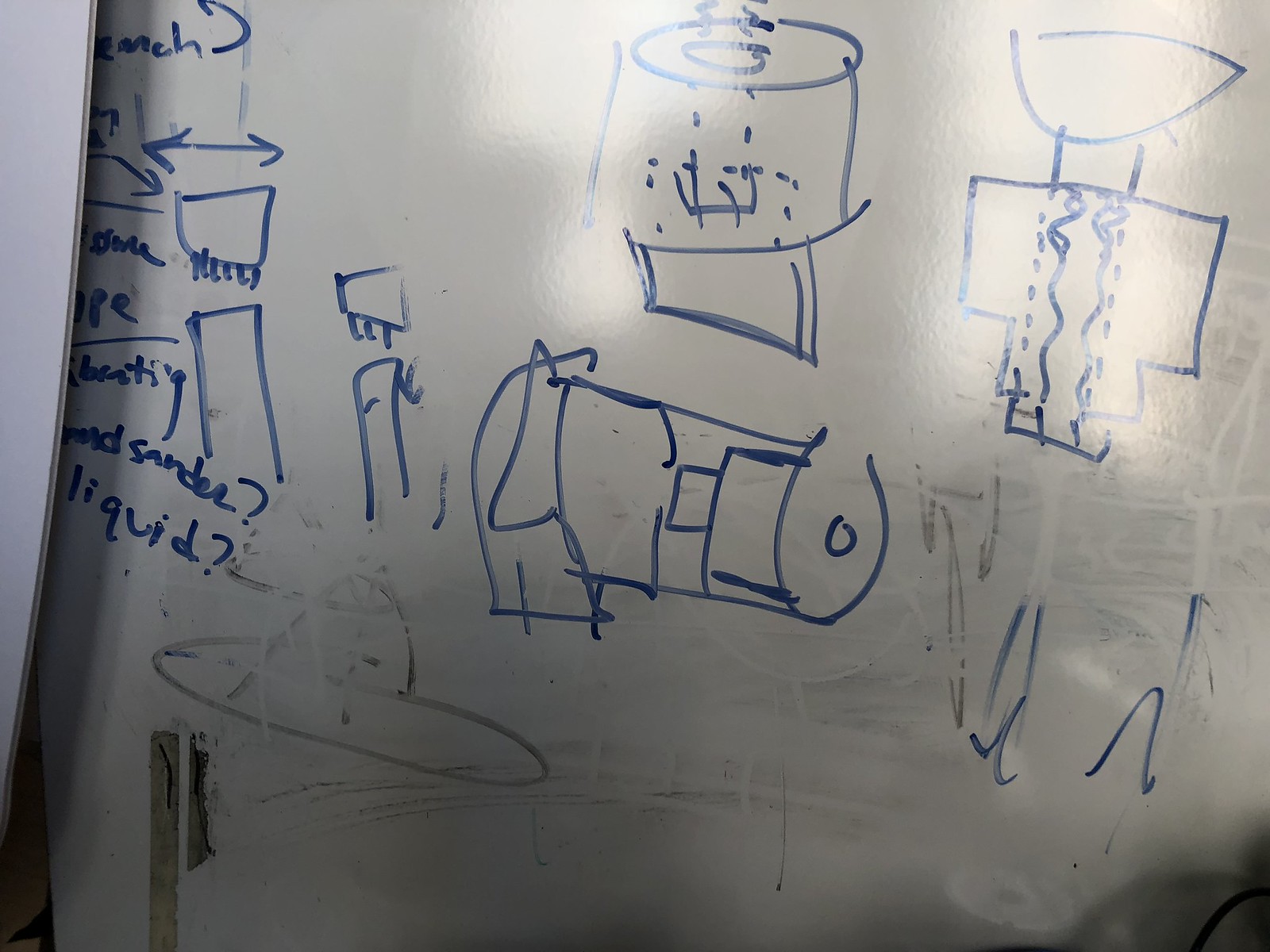This color photograph captures a whiteboard with a series of sketches and partial erasures. The textured surface of the whiteboard is evident, particularly in sections where previous drawings have been partially erased, notably near the lower portion. The remaining sketches include various shapes and unidentified figures. Legible words such as "sander," "liquid," and "vibrating" appear amidst the drawings, though some writing is partially cut off. 

An arrow, pointing both ways, connects different sections of the board, which includes multiple squares and rectangles. One sketch, resembling a hat, is primarily erased, leaving only its outline faintly visible. At the center, a cylindrical object reminiscent of a gun stands out. Above it, a rounded drawing with a circle on top and an elongated portion at the bottom evokes the image of a roll of toilet paper. 

To the right, another ambiguous figure resembles a stylized person, featuring an upside-down semicircle for a head with two lines extending downward, and a T-shaped structure that vaguely resembles a shirt. Despite the array of detailed sketches, the exact nature or purpose of each item remains unclear due to the absence of labels.